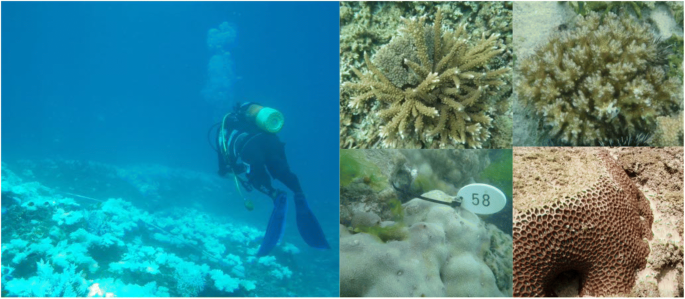The collage features five distinct images arranged on a single canvas. Dominating the left side is a large, bluish-toned photo of a person scuba diving, complete with flippers and a white tank, expelling bubbles above their head as they descend towards the ocean floor. He or she is observing diverse marine life, particularly focusing on coral formations. On the right side, four smaller images showcase various underwater scenes: lush seagrasses, different types of algae, and rocky terrains. One of these images includes a tag labeled '58,' positioned next to green seaweed. The bottom right picture displays a cliff-like structure with numerous small holes. The diver on the left seemingly captures the exquisite details presented in the adjacent four images.